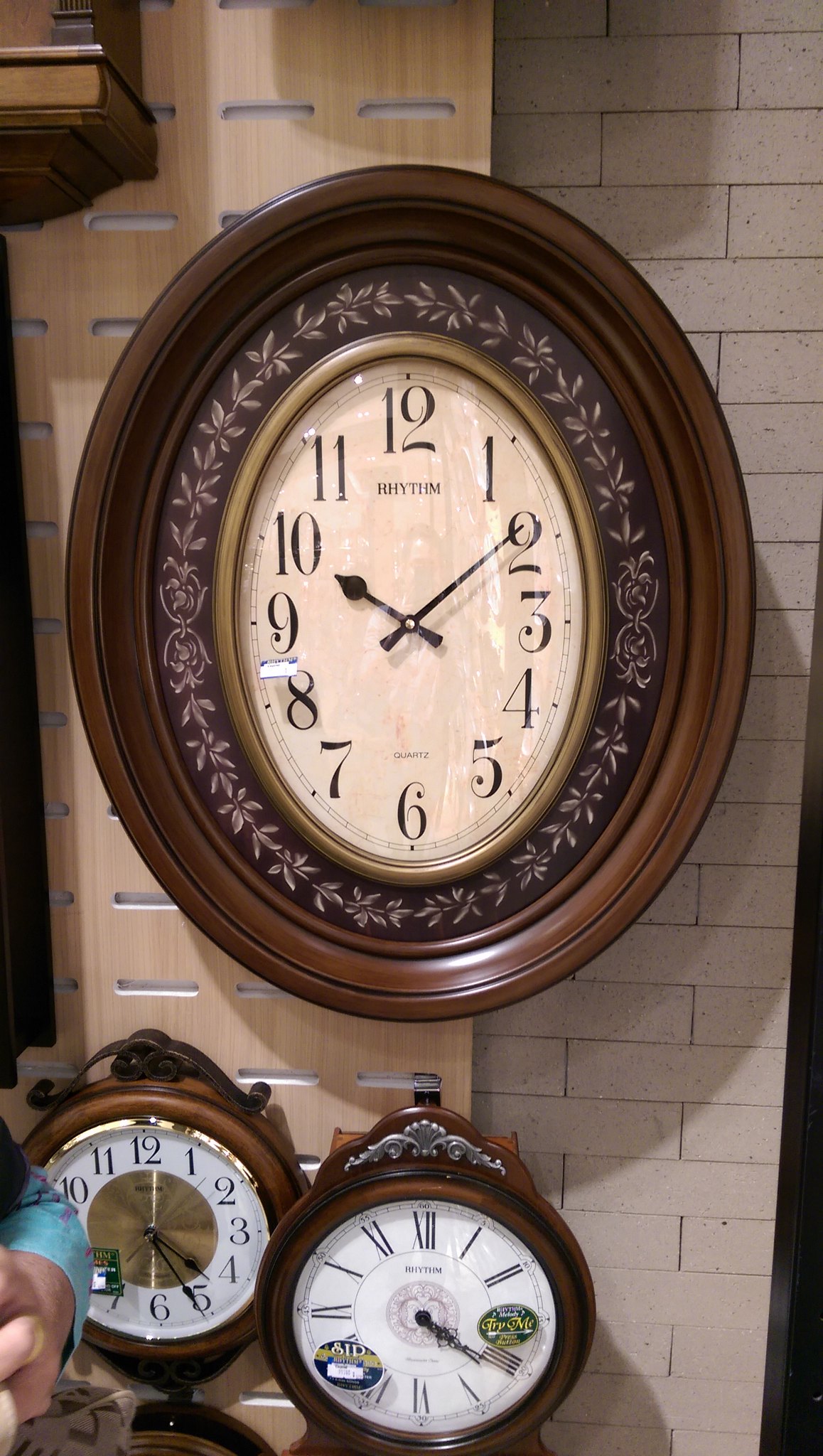The image features a trio of opulent, intricately designed clocks mounted against a backdrop that combines a white brick wall with wood paneling. The uppermost clock is encased in an oval wooden frame adorned with a floral motif, which is further accentuated by a brass oval enclosure surrounding the white dial. The clock face is marked with italic-style numerals, and the brand name "RHYTHM" is prominently displayed. The time shown is ten minutes past ten. Below this, the wall showcases two additional clocks. One of these timepieces features Roman numerals, adding a classic touch, while the other is distinguished by a brass border.